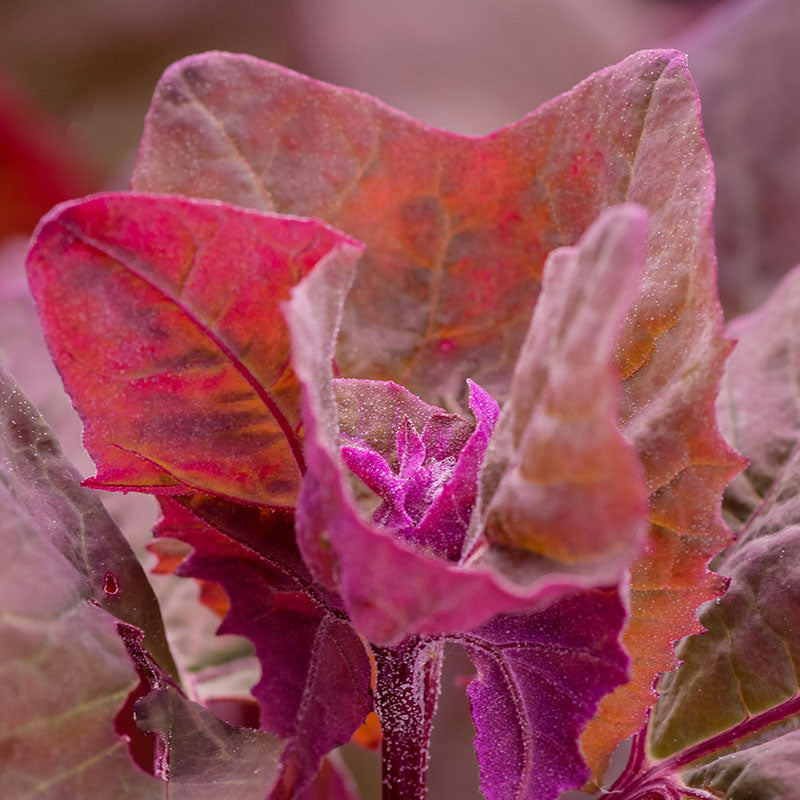This striking square-format photograph captures an extreme close-up view of a blooming plant showcasing its vibrant, multi-hued leaves. At the center of the image, a cluster of leaves exhibits shades ranging from bright magenta, pink, and fuchsia to deeper tones of red and purple, creating a stunning contrast. The central part of the plant features a tight bud, composed of small leaves in lavender tones, opening up and surrounded by brighter pinkish-red leaves with ruffled edges. A slight haze of white dust, possibly pollen, lightly obscures the vibrant colors, adding a delicate, almost ethereal quality. The background is filled with more leaves in similar hues, but they are out of focus, drawing attention to the intricate details and texture of the main cluster. At the base of this cluster, a dark purple stem provides a striking contrast to the brighter colors above, grounding the composition. The photograph merges photographic realism with a representational style, capturing the delicate beauty and complexity of the blooming plant.